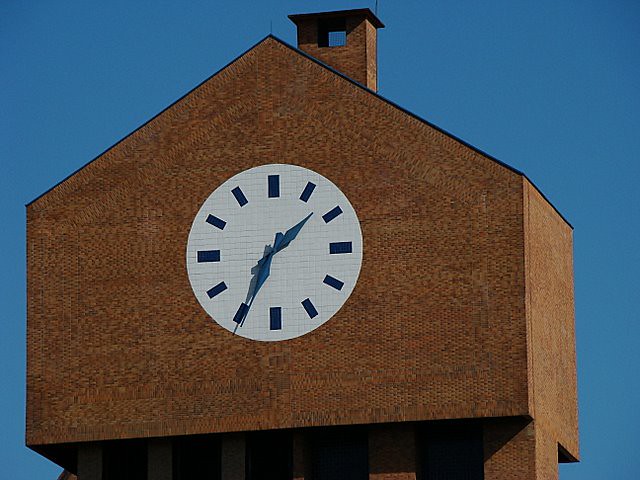This captivating photograph showcases a towering clock tower, captured from a low-angle perspective that accentuates its grandeur against a stunning bright blue sky. The edifice, constructed from red or rust-colored bricks, exudes a timeless charm with its peaked roof reaching skyward. Atop the roof, a distinctive rectangular chimney adds architectural interest, featuring an open square that frames a slice of the azure heavens beyond. Central to this magnificent structure is the clock face itself—a pristine white, circular design prominently positioned on the brick facade. Unique rectangular shapes mark the hours from 1 through 12, offering a modern twist on traditional numerals. This harmonious blend of historical and contemporary design elements is further highlighted by the vivid clarity of the sky, making for a visually arresting image.